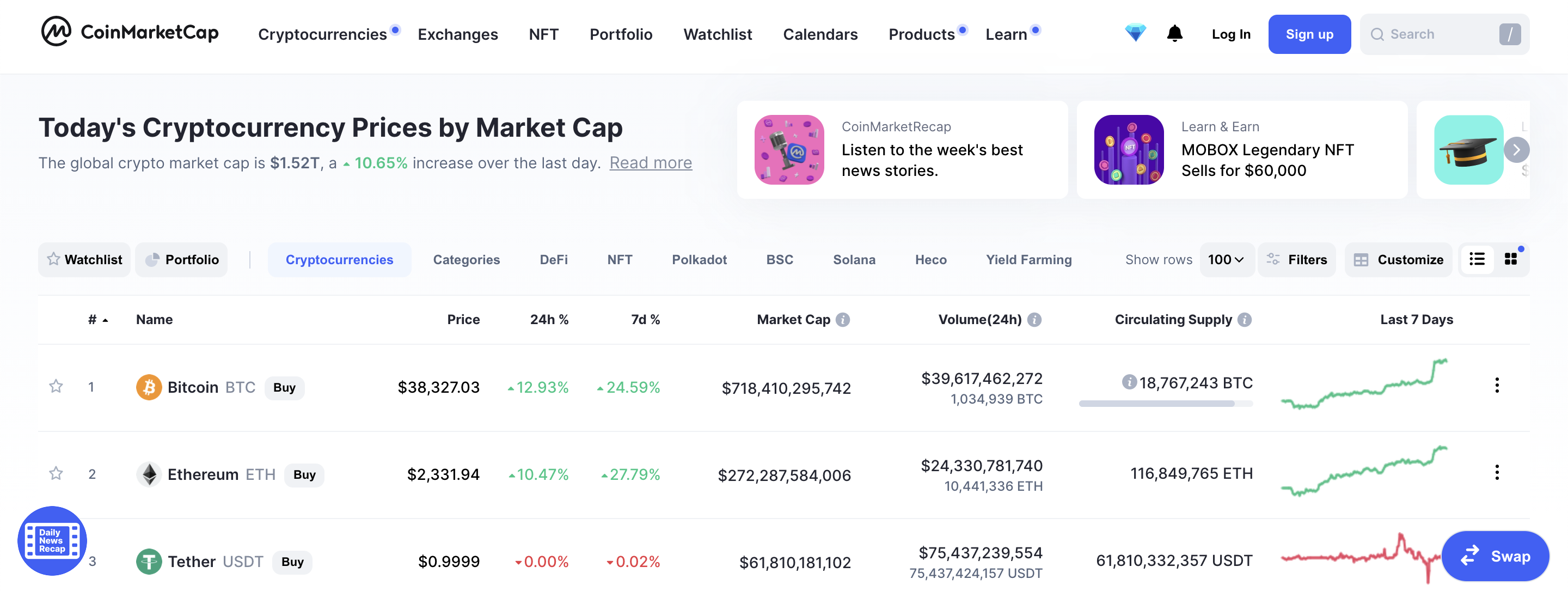Today's Cryptocurrency Market Update: Bitcoin is currently priced at $38,000, while Ethereum stands at $2,230 and Tether at $0.9999. Explore the week's top news stories in the cryptocurrency world. Stay updated with CoinMarketCap for information on various cryptocurrencies, exchanges, and NFTs. Manage your portfolio with tools like watchlists and calendars. For more in-depth knowledge, check out our products and learning resources. Log in or sign up to swap and access more features.